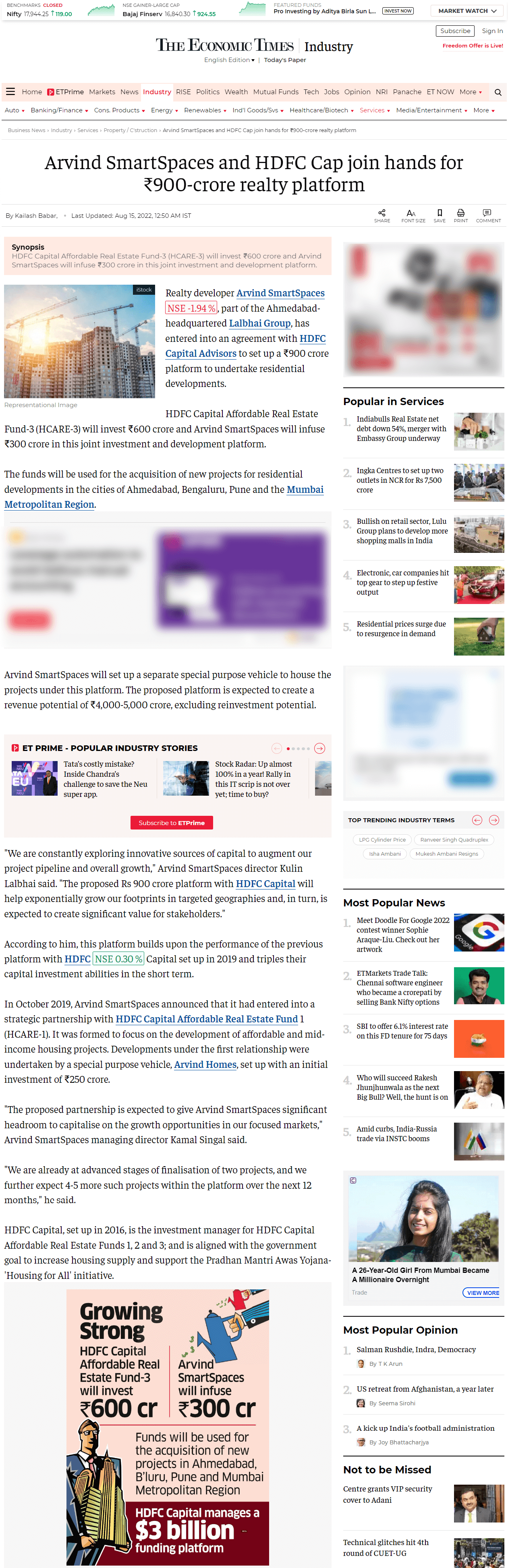The image captures a headline from The Economic Times Industry section. At the top, the title is prominently displayed. Below the title is a long pink line with very small, unreadable text within it. In bold black text, the headline reads: "ARVIND Smart Spaces and HDFC Cap Join Hands for ₹900 Crore Realty Platform." The background of the image features an array of tall, gray buildings set against a bright sky, indicating either sunrise or sunset. Scattered sections of very small, unreadable text occupy the lower portion of the image. In a square at the very bottom, the phrase "Growing Strong" is displayed next to the image of a man in a suit. Beside this, there is a figure indicating "₹3 billion." In the upper right corner of the pink line, an arm extends holding a watering can, with water sprinkles coming out. Additionally, to the right, the image of a smiling woman with dark hair, standing in front of a picturesque mountain range, is visible.